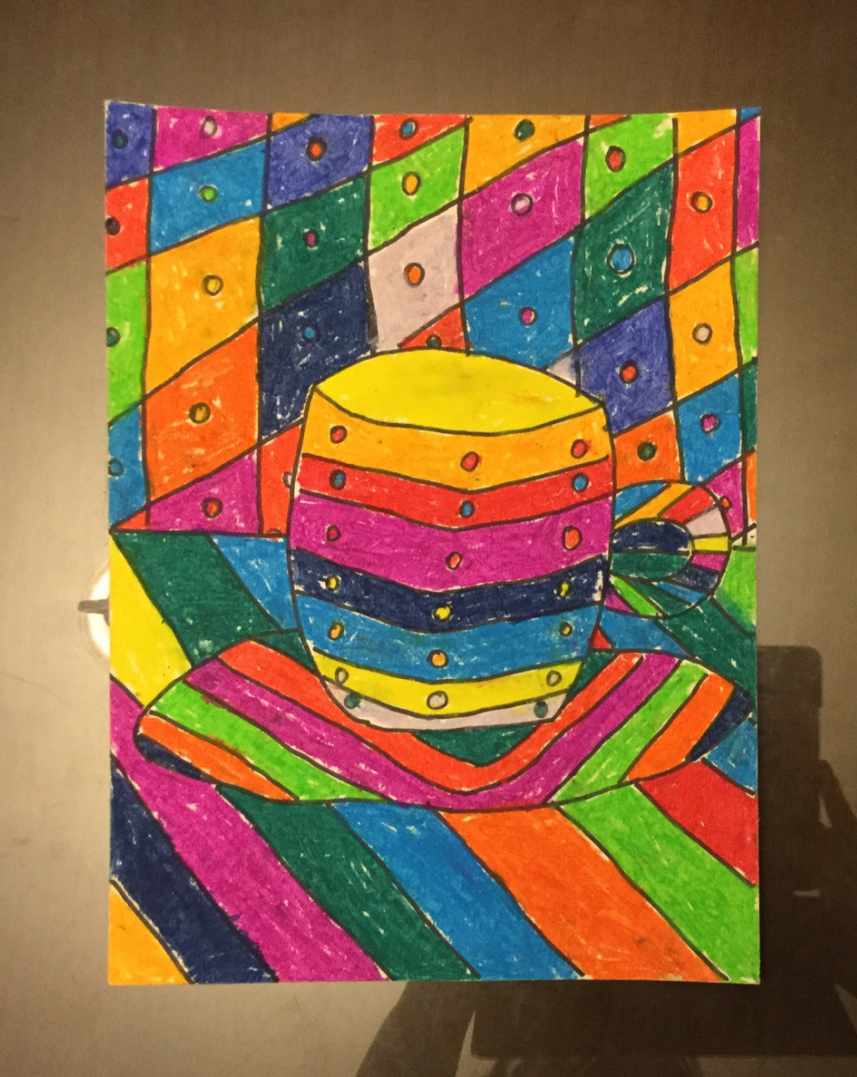This photograph captures a mesmerizing piece of multicolored artwork, displayed on what appears to be a glass table. The reflective surface of the table showcases a light source in the upper left corner, enhancing the vibrant colors of the artwork. In the bottom right-hand corner, a subtle shadow reveals the presence of the photographer, likely using an iPad, with the faint silhouettes of their arms, fingers, and a portion of their head visible.

The artwork itself is an explosion of color, where every inch of the canvas is meticulously adorned. The background features a captivating diagonal diamond grid interspersed with playful polka dots. The bottom half of the piece transitions into vivid rainbow stripes, creating a lively foundation for the central subject. Nestled on this bed of colors is a whimsical, rainbow-colored saucer with a matching coffee cup perched neatly atop it. This striking combination of patterns and hues creates a visually stunning and dynamic composition.